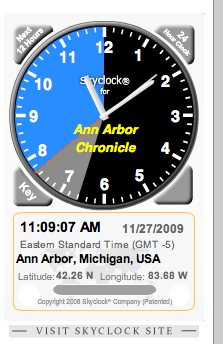The image, set against a white background with a gray vertical line on the right, prominently features a round clock with Arabic numerals and hash marks for minutes. The clock face is divided into three distinct colored sections: a blue area on the left taking up about one-third, a smaller gray strip below it, and a black section occupying the right. The text "Ann Arbor Chronicle" is displayed in light yellow below the clock's center. Triangles with arrows and labels point from various corners to parts of the clock: an arrow in the upper left labeled "Next 12 hours", an upper right arrow labeled "24 hour check", and a lower left arrow labeled "Key" with the lower right triangle remaining unlabeled. The clock shows the time stopped at 11:09:07 AM with the second hand at approximately 8 seconds, dated 11.27.2009 Eastern Standard Time. Beneath the clock, a block of black text reads "11:09.07am 11.27.2009 Eastern Standard Time GMT-5 Ann Arbor, Michigan Latitude 42.26 North Longitude 83.68 West", followed by "Copyright 2008 SkyClock Company Patent" and an invitation to "Visit SkyClock site".